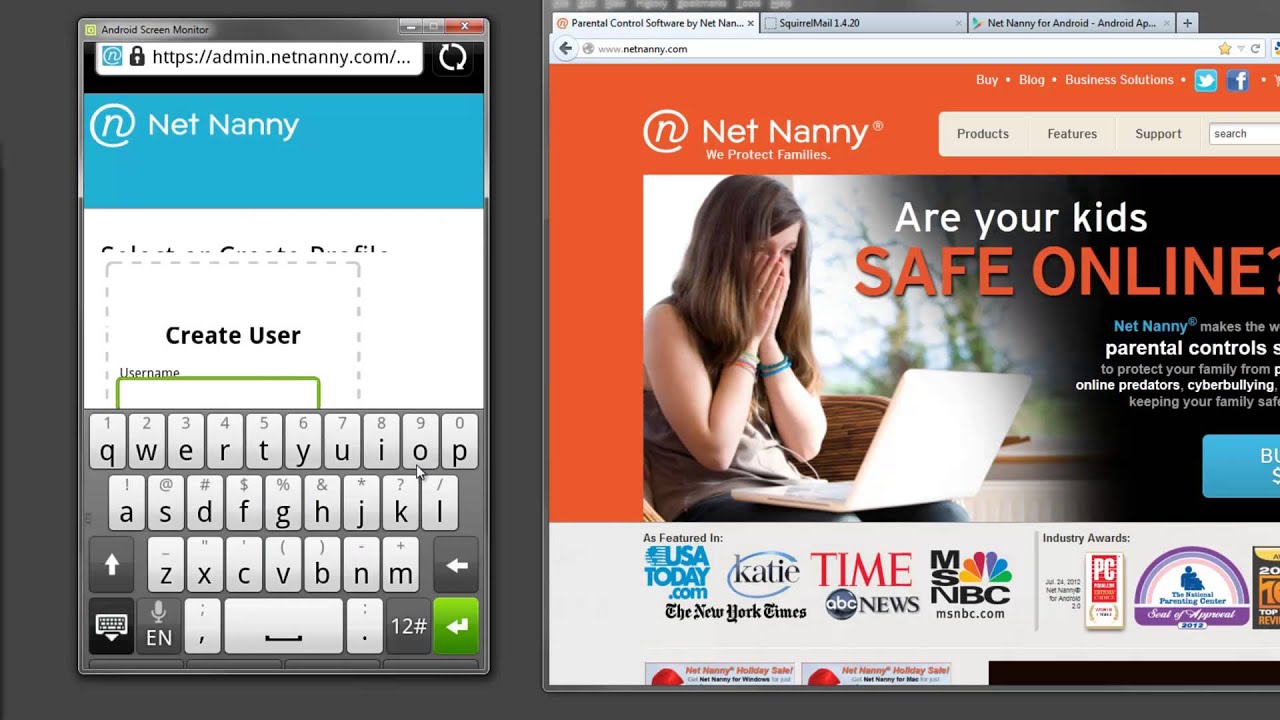This rectangular image is divided into two distinct sections: a website interface on the left and a web page featuring a woman on the right, all set against a gray background.

On the left side of the image, the web page has a URL at the top reading "https://admin.netnanny.com/...". To its right, a white refresh icon is visible. Directly below the URL, the text "Net Nanny" is displayed, followed by the phrase "Create User." Below this, there is a clear indication for "Username," accompanied by a rectangular green-bordered input box intended for entering user credentials. Beneath this input box, an on-screen keyboard with alphabet letters is visible, presumably for entering the username.

The right side of the image features a photograph of a woman who is captured in a moment of surprise or shock, with both of her hands covering her mouth. She is sitting down with a laptop resting on her lap, suggesting she is reacting to something on the screen in front of her.